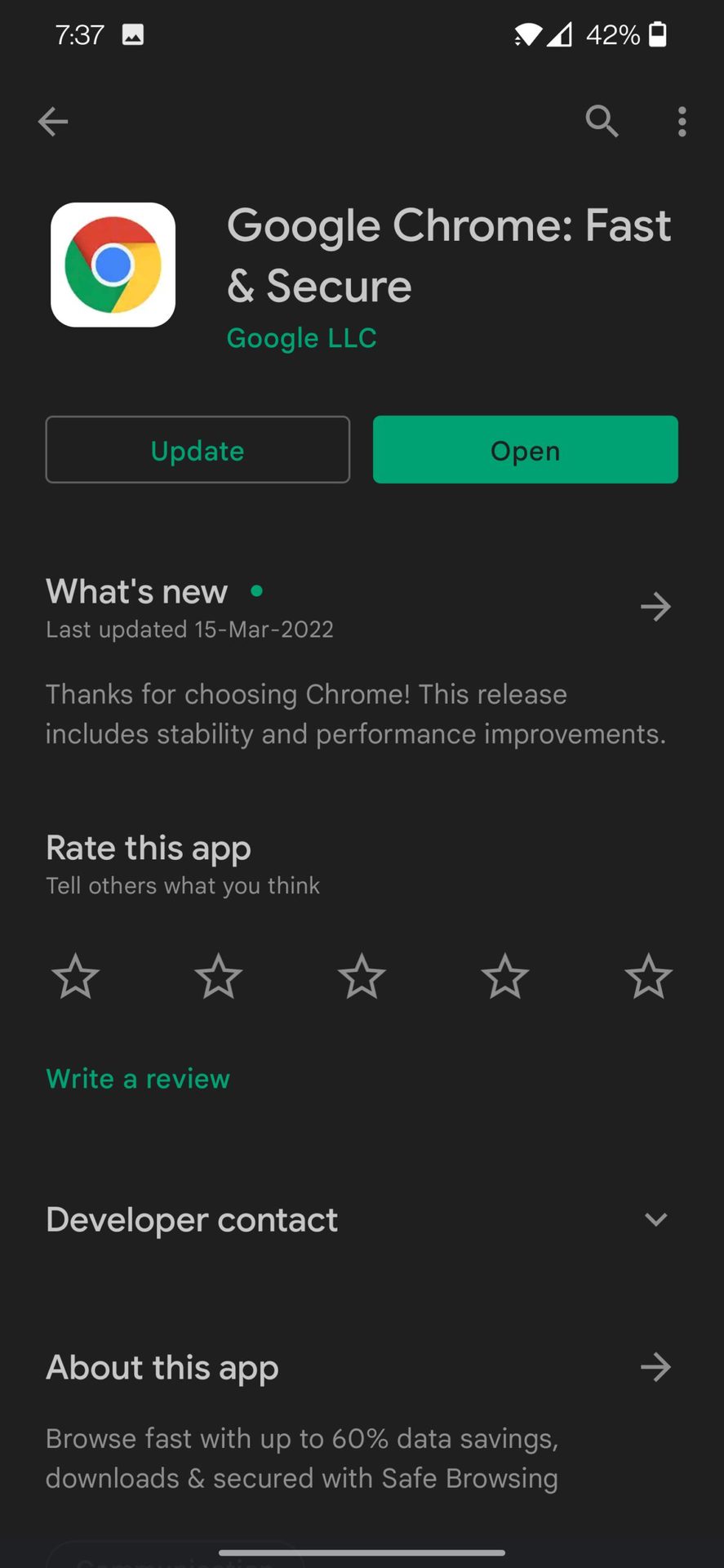This image displays the Google Play Store app on a smartphone with a sleek black background. At the forefront is the listing for the "Google Chrome: Fast & Secure" app. The prominent Google Chrome icon, featuring a circular design with green, red, blue, white, and yellow colors, is placed at the top left corner against a white background. Below the app's name, "Google LLC" is written in green text.

In the middle segment of the screen, two functional buttons are displayed: "Update" on the left, written in green with a black background, and "Open" on the right, written in black with a green background. 

Further down, the section titled "What's New" notes that the app was last updated on 15 March 2022. The accompanying text reads, "Thanks for choosing Chrome. This release includes stability and performance improvements."

At the bottom, there's an invitation to "Rate this app, tell others what you think" followed by five unrated, grey stars. Beneath these stars, green text encourages users to "Write a review." Below this, additional white text provides a link to "Developer contact" and lists key app features: "About this app, browser fast, up to 60% data savings, download and secure with safe browsing."

Overall, both the app interface and the background maintain a consistent black theme, enhancing the contrast and readability of the text and iconography.